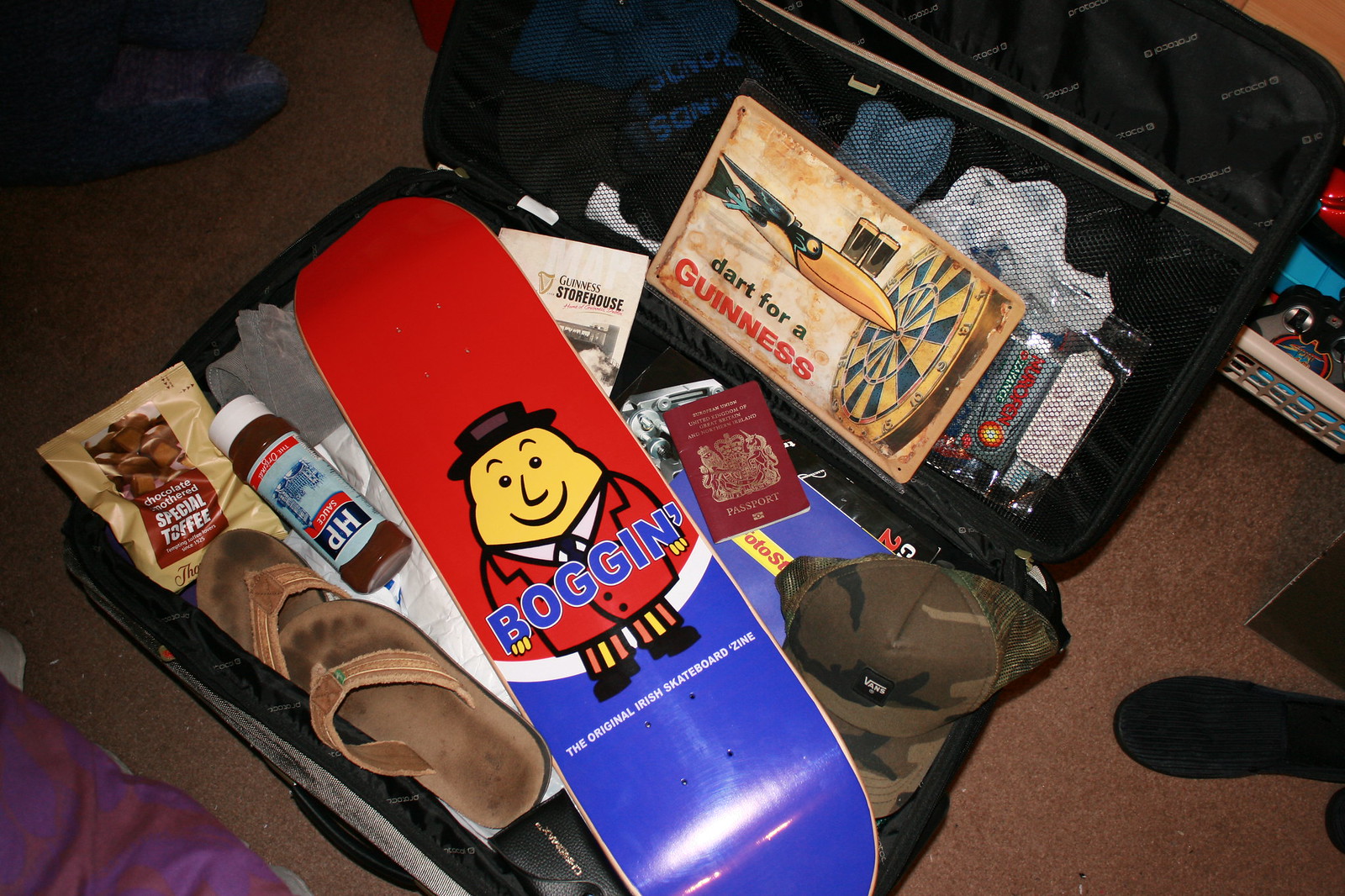This photograph captures the interior of an open black suitcase, showcasing an eclectic assortment of items meticulously packed. Dominating the center of the suitcase is a uniquely designed board, likely a skateboard or a snowboard. The board features a vibrant design, with a red top and a contrasting blue bottom, connected by a curving white line. Prominently displayed on the board's surface is a quirky cartoon character with a lumpy yellow head, black eyes, and a black smile, donning a small top hat, red jacket, white collared shirt, dark black tie, and red-yellow striped pants. Positioned above the character is the text "Boggin," styled in blue with a white outline, accompanied by the tagline "the original Irish skateboard zine," emphasizing its unique cultural backstory.

Surrounding the board are various items, adding depth to the suitcase's contents. At the top left, a cream-colored packet of toffees marked "special toffee" catches the eye. Adjacent to it, an inverted HP Sauce bottle with a blue label and white cap sits beside some well-worn brown sandals, complete with visible foot marks. A British passport, with its distinguishing red cover and gold emblem, lies nearby along with a booklet from the Guinness Storehouse. Additionally, a camouflage hat emblazoned with the Vans logo and an old postcard or sign featuring a toucan with Guinness pints balanced on its beak and a clever "Dart for a Guinness" slogan contribute to the rich visual narrative. The suitcase's netted compartment holds some tablets, hinting at practical necessities, while scattered clothes enhance the scene. All this is set against the backdrop of a brown carpet around the suitcase, completing the detailed tableau.